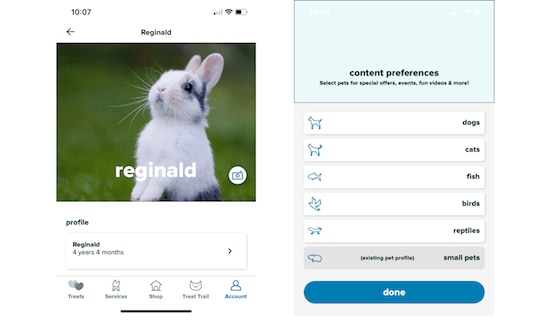The image depicts the screens of two mobile devices side by side. 

### Left Screen:
- **Top section**:
  - Displayed time: **10:07 AM** located at the top left corner.
  - Status icons at the top right corner: signal bars for cellular network, Wi-Fi signal, and a half-full battery icon.

- **Main Display Area**:
  - **Header**: Contains a left-pointing arrow.
  - **Title**: Centrally displayed text reading "Reginald" in bold letters.
  - Below the title is an image of a white bunny with distinctive black markings. The bunny is perched on its hind legs with its front legs raised off the ground.
  - Below the image, the bunny's name "Reginald" is displayed again in white text within a green field, though the field appears slightly blurry.
  - At the bottom right corner of the image is a circular icon featuring a camera, labeled "Profile".
 
- **Additional Information**:
  - A label: "Reginald, four years, four months" followed by a right-pointing arrow.

- **Menu Options**:
  - Listed below the additional information are tabs reading: Treats, Services, Shop, [Something], Trail, and Account.

### Right Screen:
- **Content Categories**:
  - A header with the title: "Content Preferences".
  - Subtitle: "Select Pets for Special Offers, Events, Fun, Videos and More".
- **Category List**:
  - **Pets**:
    - Dog
    - Cat
    - Fish
    - Birds
    - Reptiles
    - Small Pets
  
  - Each pet category features black text with corresponding blue icons on the left side.

These details combine to offer a comprehensive view of the mobile device interfaces, likely within a pet management or pet-themed application.